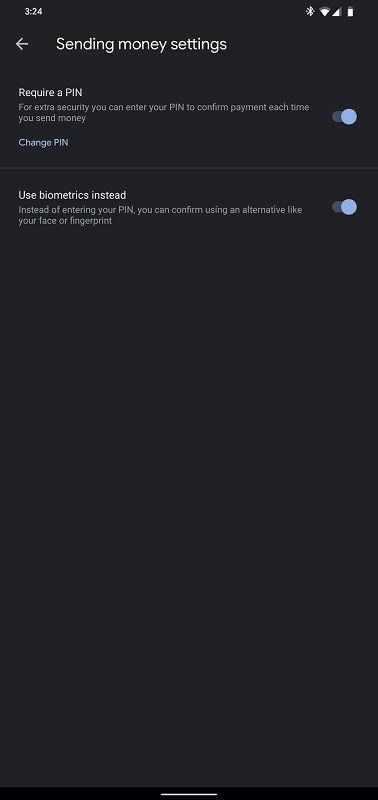The image depicts a mobile phone screen with a black background. In the upper left corner, the time is displayed as 3:24. Beneath the time, a small white arrow points left, followed by the text "Sending Money Settings."

The first section is labeled "Require a PIN." In very small white text below this label, it reads, "For extra security, you can enter your PIN to confirm payment each time you send money." To the right of this text, there is a blue toggle circle.

Underneath is an option labeled "Change PIN."

The next section, in white text, is titled "Use Biometrics Instead." Below this title, the text explains, "Instead of entering your PIN, you can confirm using your face or fingerprint." Next to this section, there is another blue toggle circle positioned to the right.